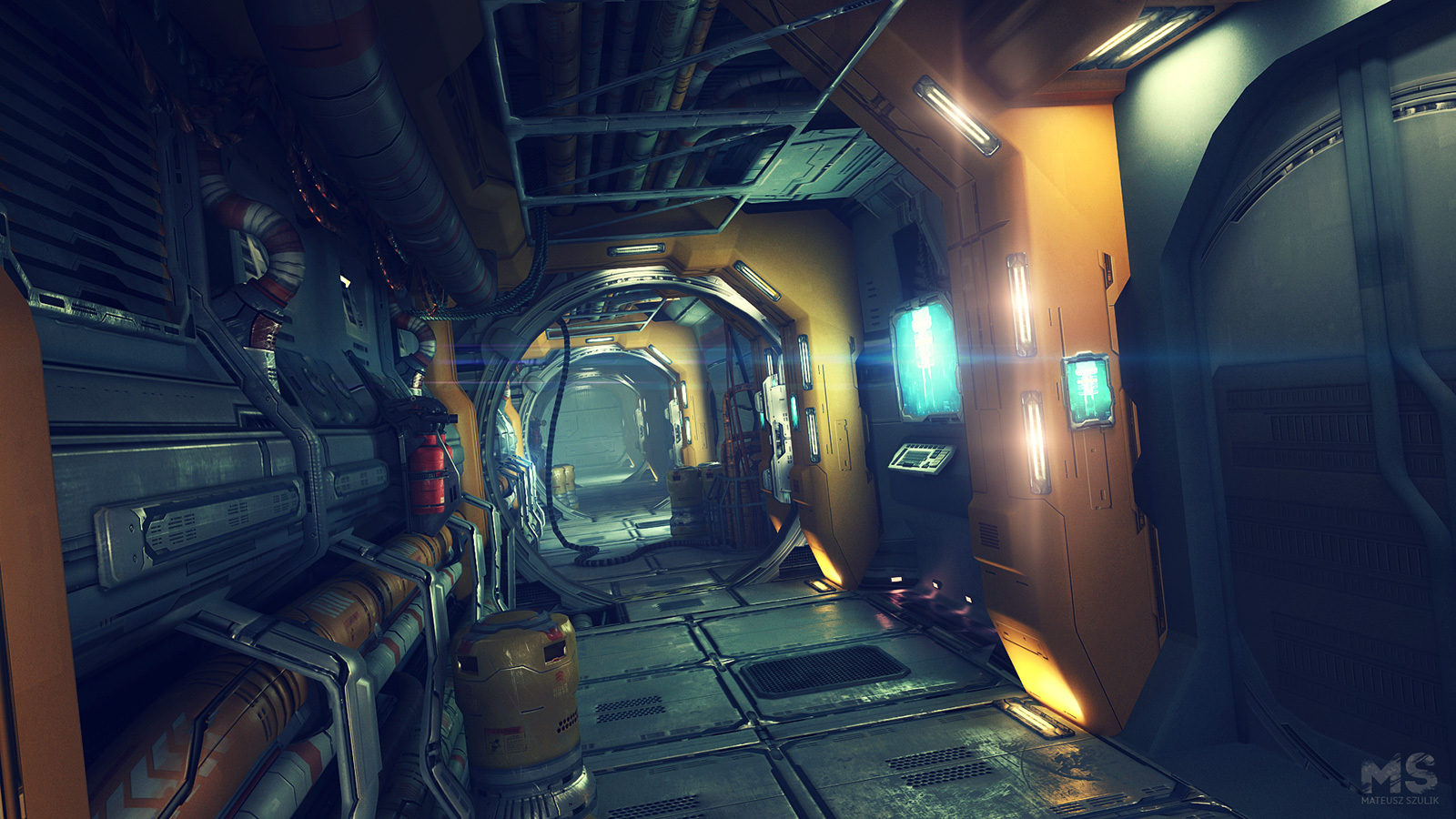The image depicts a detailed, computer-generated interior of a spaceship, evocative of scenes from a science fiction movie or video game. Dominated by dark brown and green hues, the scene highlights a long corridor with round bulkheads that could be doors, lined with various pieces of intricate equipment and tanks. The floor is tiled with hatches, some featuring vents, and a hose snakes across it, lying beside several barrels. Numerous lamps illuminate the hallway, casting light on key elements such as a computer terminal positioned center-right, displaying an image that is mirrored on a tablet mounted next to a nearby door. Above the tablet, white lights add to the futuristic ambiance. In the lower right corner of the image, the initials 'MS' are inscribed next to the name 'MATEUSZ SZULIK,' suggesting this may be a screenshot from a PC game.